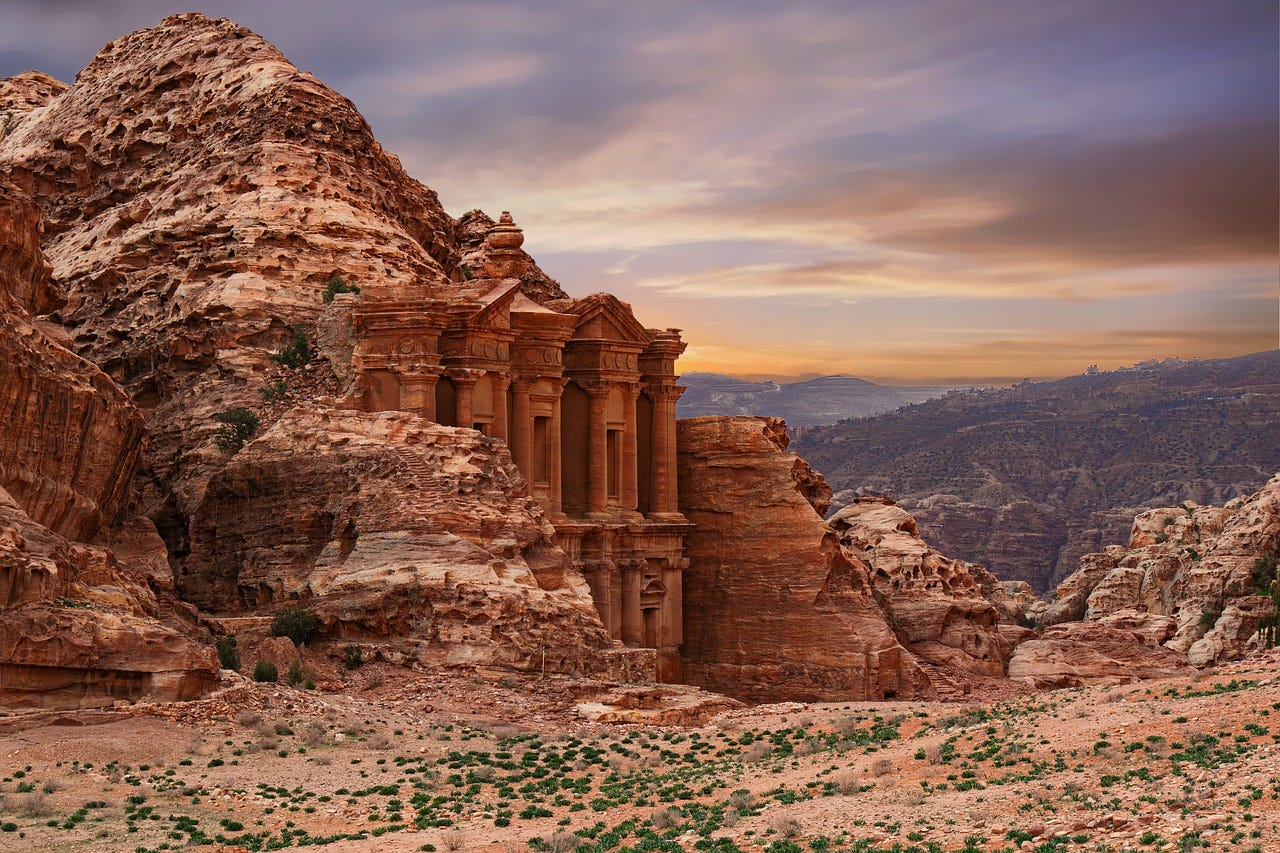The photograph captures an arresting, rugged landscape dominated by a jagged and uneven rock face that features intricate ancient ruins carved into its central area. The rocky facade displays a spectrum of rust and iron ore tones, ranging from light browns and beiges to darker shades, often arranged in horizontal sections. The ruins, partially obscured, resemble multi-story stone pillars and columns, with large circular designs stacked atop each other.

Below the rock face spreads a flat expanse of reddish gravel interspersed with sporadic, short tufts of dark green grass. In the background to the right, a range of darker, less jagged mountains provides a stark contrast to the varied terrain in the foreground. The top third of the photograph showcases a dramatic sunset, with wispy dark blue, grey, and white clouds illuminated by a thin strip of yellow as the sun begins to set. This scene merges the ancient with the natural, painting a vivid picture of enduring historico-geological beauty.